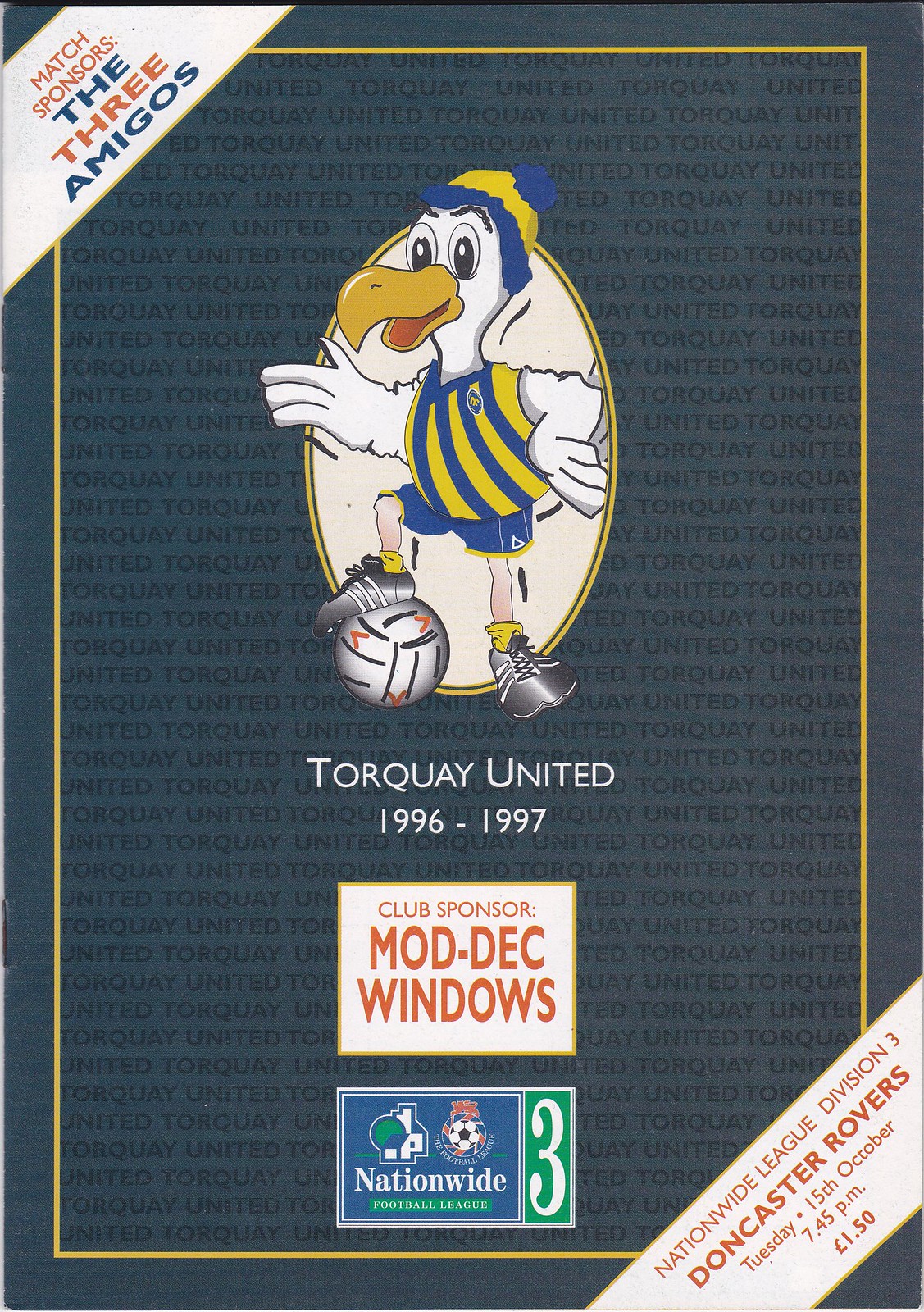The front cover of this magazine features a striking image of a cartoon duck mascot standing confidently with one foot on a soccer ball. The duck is adorned with a blue and yellow striped beanie, a matching yellow and blue striped shirt, blue shorts, and gray cleats. His left wing is extended outwards while his right rests on his hip. Centered within an oval background, the mascot's uniform highlights the vibrant team colors.

Above the mascot, the logo of Torquay United from the 1996 to 1997 season is prominently displayed. The cover is framed by a gold rectangular border, set against a dark blue background that is repeatedly inscribed with the team's name. Below the mascot, in white text, it reads "Torquay United 1996-1997," followed by two rectangular boxes. The first, stating "Club Sponsor ModDeck Windows," and the second, "Nationwide Football League."

Additionally, the upper left corner features a diagonal banner with the text "Match Sponsors The Three Amigos." Meanwhile, the lower right corner includes another banner detailing "Nationwide League Division 3, Doncaster Rovers, Tuesday 15th, October 7:45 p.m., £1.50."